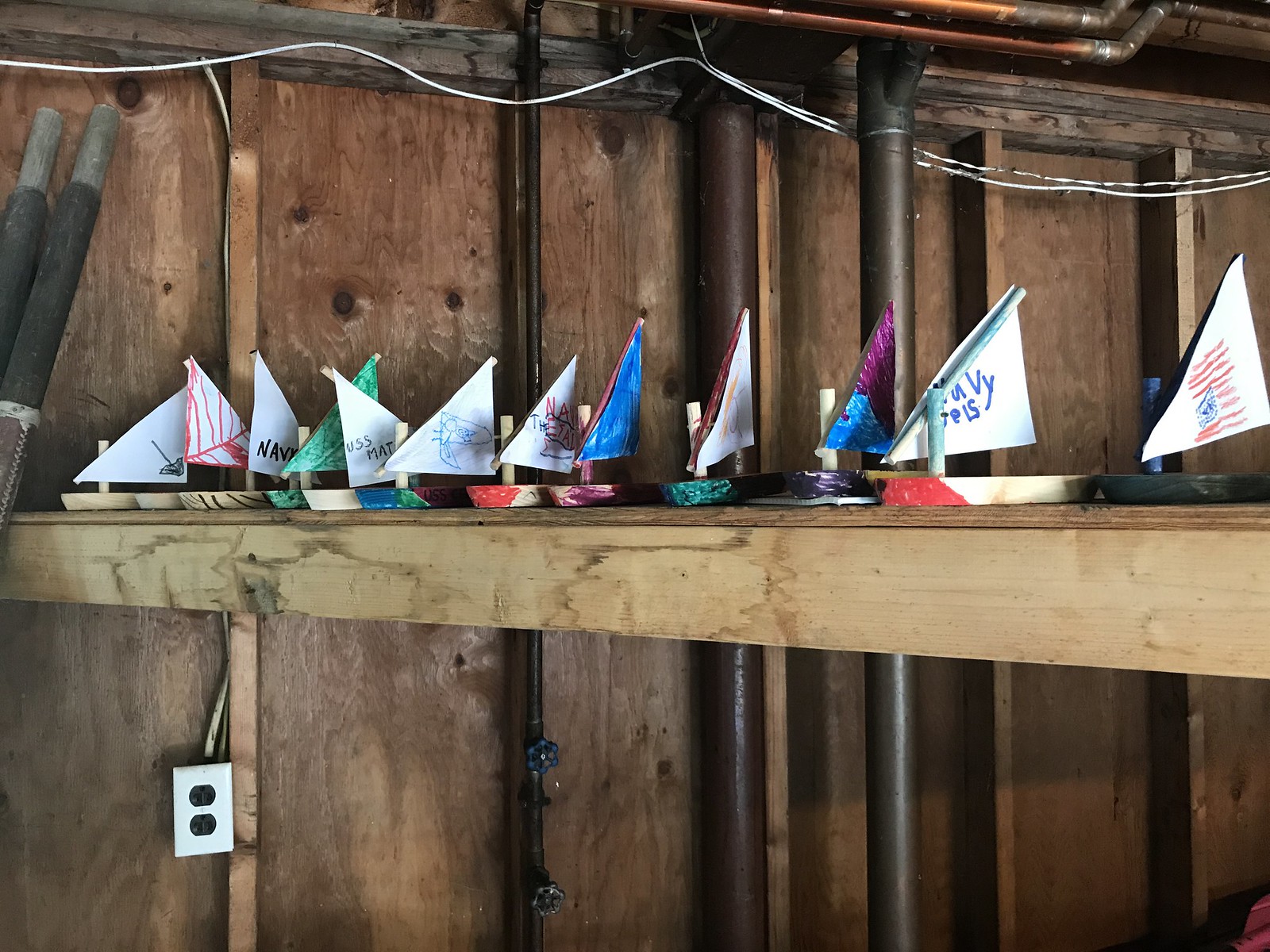In this photograph, an indoor scene depicts an unfinished wooden shed or basement area. The backdrop consists of unpainted dark brown plywood walls, accented with vertically oriented grayish two-by-four studs and accentuating copper pipes winding up to the top right section. Various dark gray and dark brown pipes cascade downward on the right side, and an electrical outlet with a black faceplate is fixed to one of the two-by-fours on the lower left. In the top left corner, two dark gray poles stand against the frame, while white electrical wires dangle from the ceiling.

The central wooden beam, stretching from the left to the right side of the image, serves as a whimsical display for approximately twelve small, handcrafted sailboats. These miniature boats feature wooden bases and colorful paper sails, likely adorned with markers or crayons, indicative of a children's craft project. The sails exhibit a spectrum of hues including blue, red, green, and purple, with some distinctly marked with words like "Navy" and "USS Matt." These toy sailboats vary in simplicity but uniformly face a single direction, creating a sense of coherence amidst the rustic, utility-filled setting.